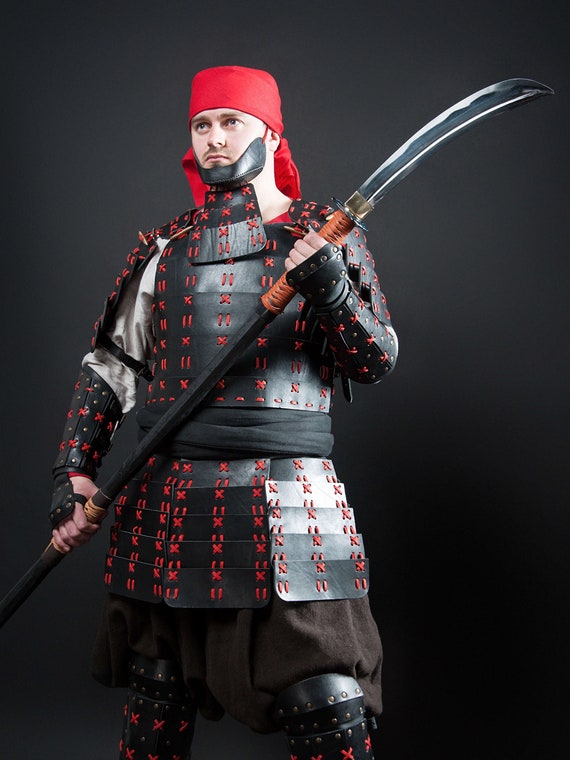The image portrays a young white man dressed in detailed, cultural Japanese armor reminiscent of the Sengoku era. The armor, made from various leather plates stitched together with striking red thread in patterns resembling Xs and dashes, covers his torso and extends to protective sections around his legs. He dons a red bandana and a leather chinstrap, adding to the authenticity of his appearance. His hand grips a formidable staff with a machete blade at its end, reflecting traditional Japanese weaponry. The entire ensemble includes hand protectors and a black band around his waist, enhancing the overall ceremonial look. The lighting in the image comes from the right side, illuminating his leftward gaze against a stark, empty black background. This intricate getup might suggest he is a cosplayer, meticulously emulating historical Japanese warriors with handmade precision.